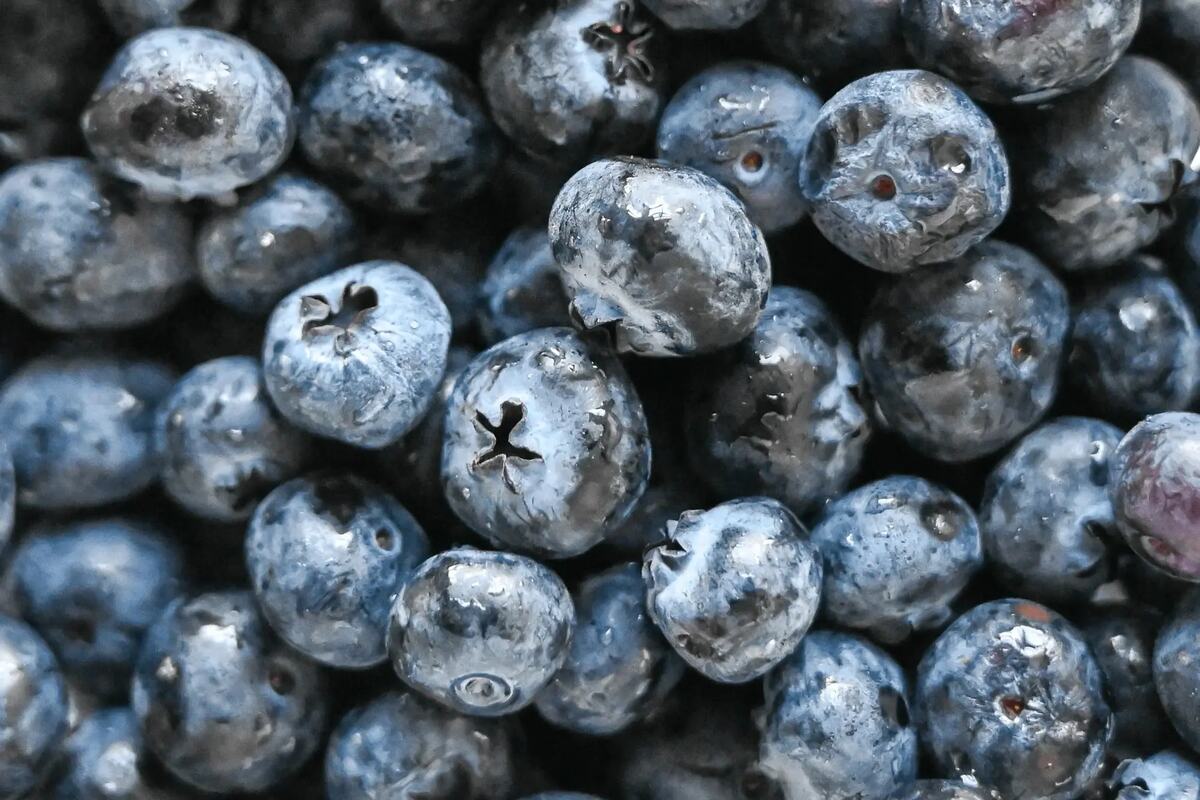This rectangular photograph captures a close-up view of roughly 30 to 40 small, round fruits that strongly resemble blueberries. The fruits are predominantly dark in color, ranging from black to deep blue. Their surfaces display a mix of white and light brown patches, possibly indicative of natural variations or some form of coating, which suggests they might be jamun or blueberries. Some of the fruits are adorned with delicate water droplets, indicating the freshness and cleanliness of the fruit. Light reflects softly off their smooth, glossy surfaces, suggesting that the picture was taken indoors, under controlled lighting conditions. The arrangement of the fruits appears random, creating a natural and abundant look, akin to a bushel of freshly gathered berries ready for consumption.